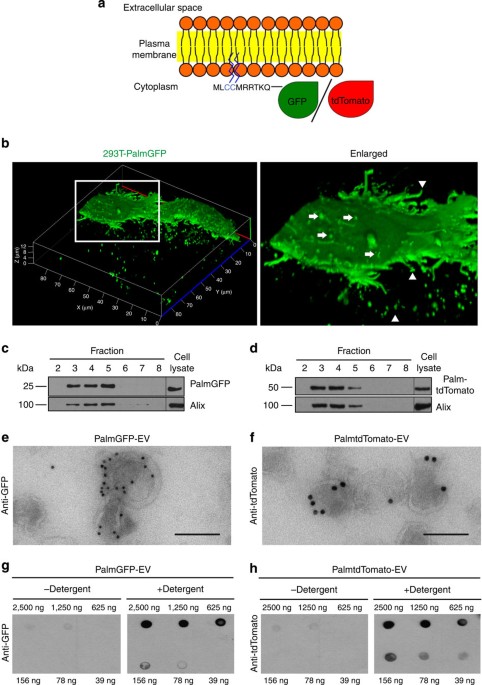The image is a detailed scientific chart against a white background, organized into sections labeled A through H. At the top (Exhibit A), there is a labeled diagram showing the extracellular space, plasma membrane, and cytoplasm. This section features interconnected rows of orange balls illustrated in yellow strips and includes depictions labeled GFP in green and 'Tomato' in red.

Beneath this, Exhibit B displays thermal-like imagery with a black background, featuring bright neon green formations labeled '293 T palm GFP.' An enlarged version of this green image is also shown. Sections C and D consist of charts representing fractions one through eight, alongside a meter indicating 'cell lysate.' 

Sections E and F include grayscale diagrams with black specks labeled 'palm GFP-EV' and 'palm TD tomato-EV,' respectively. Finally, sections G and H show gray diagrams with numerical labels '25,000 NG,' detailing 'minus detergent' and 'plus detergent' scenarios for 'palm GFP-EV' and 'palm tomato-EV.' 

Overall, the image seems to illustrate various cellular components and conditions, potentially connected to plant biology, with specific focus on GFP and 'Tomato' markers.